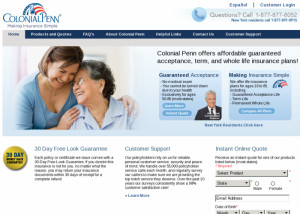The website for Colonial Penn is prominently displayed, inviting visitors to explore their insurance offerings. Colonial Penn has long been recognized, primarily through iconic TV commercials, for providing life insurance targeted at seniors, aiming to help cover funeral expenses and alleviate financial burdens on loved ones. Notably, since the era of Bob Barker on "The Price is Right" in the 70s, Colonial Penn's advertisements have been a mainstay. 

The website proudly features a picture of Alex Trebek, the esteemed host of "Jeopardy!", who once endorsed Colonial Penn. To the left of this image is a touching photograph of a daughter hugging her mother, creating an emotional appeal and reassurement for users that "everything is going to be alright."

Further down, the site outlines their offerings in three clear columns: a 30-day look-over guarantee, dedicated customer support, and instant online quotes, allowing potential customers to easily explore their insurance options.